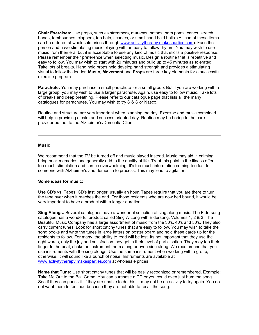This image is a low-quality screenshot of a document, making it challenging to decipher any meaningful content. The text appears as blurred, indistinct shapes, likely due to the excessive zoom and poor resolution. The document consists of several paragraphs: three are located at the top with a noticeable blue hyperlink embedded within the first paragraph. A dividing line separates these from the bottom section, which possibly features a header or title. Below this header are four additional paragraphs, with the third one containing another blue hyperlink. The text is rendered in black on a white background, but the characters are too pixelated to determine whether they are in English or another language.